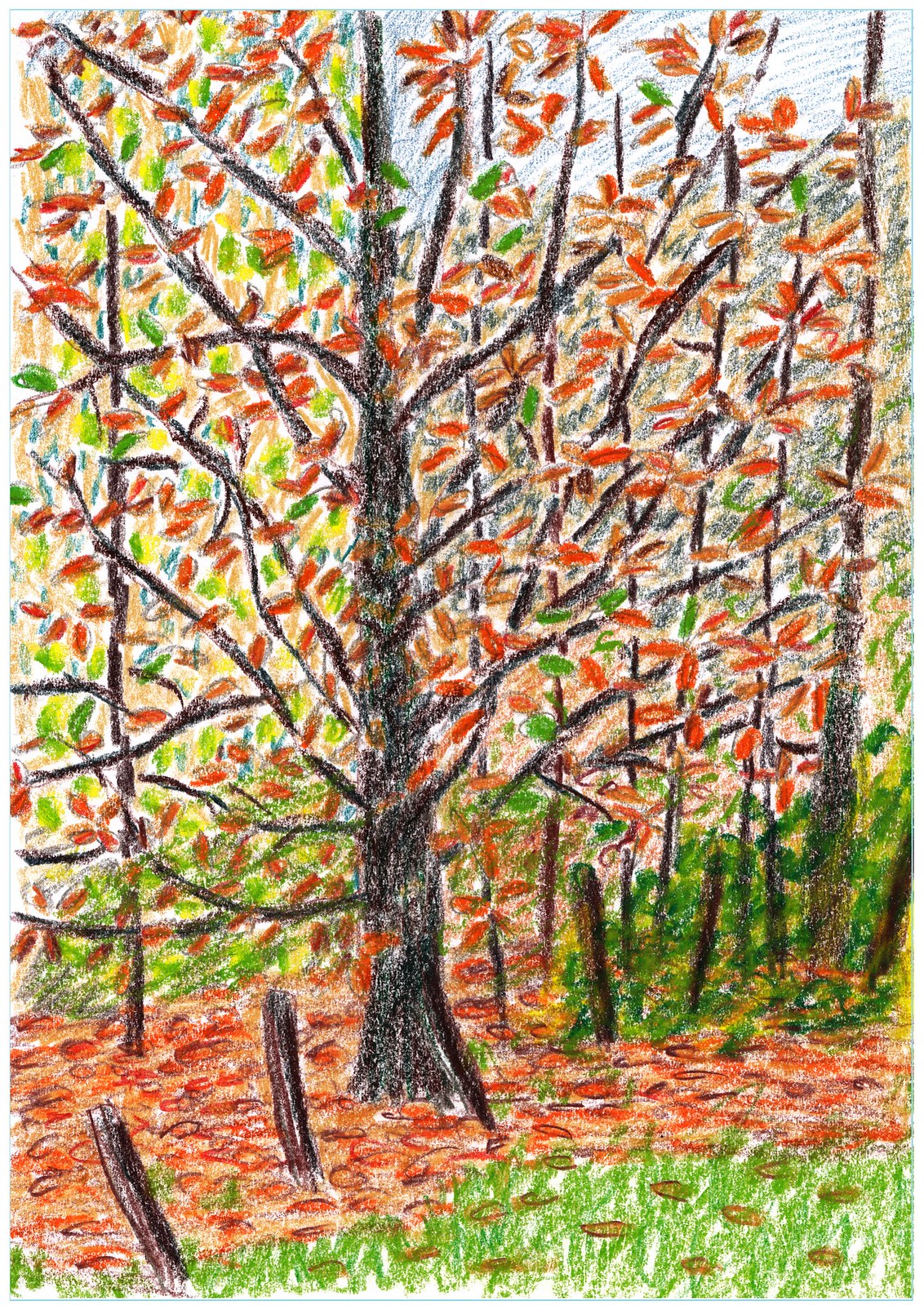This colored pencil drawing beautifully captures the serene ambiance of an autumnal landscape. At the center, a large tree stands proudly, its leaves transitioning to a vivid yellow, indicative of fall. Several of these golden leaves have gracefully descended to the ground, forming a delicate carpet over the still predominantly green grass. The area directly surrounding the tree showcases a blend of green grass and scattered fallen leaves. Adjacent to this tree are subtle indications of other trees, some retaining their green foliage in contrast with the yellowing leaves of the central tree. Branches extend skyward, adding texture and depth to the composition. In the bottom right corner, a bush contributes to the scene's lush vegetation. Above, a portion of the blue sky peeks through, completing this tranquil autumnal tableau.